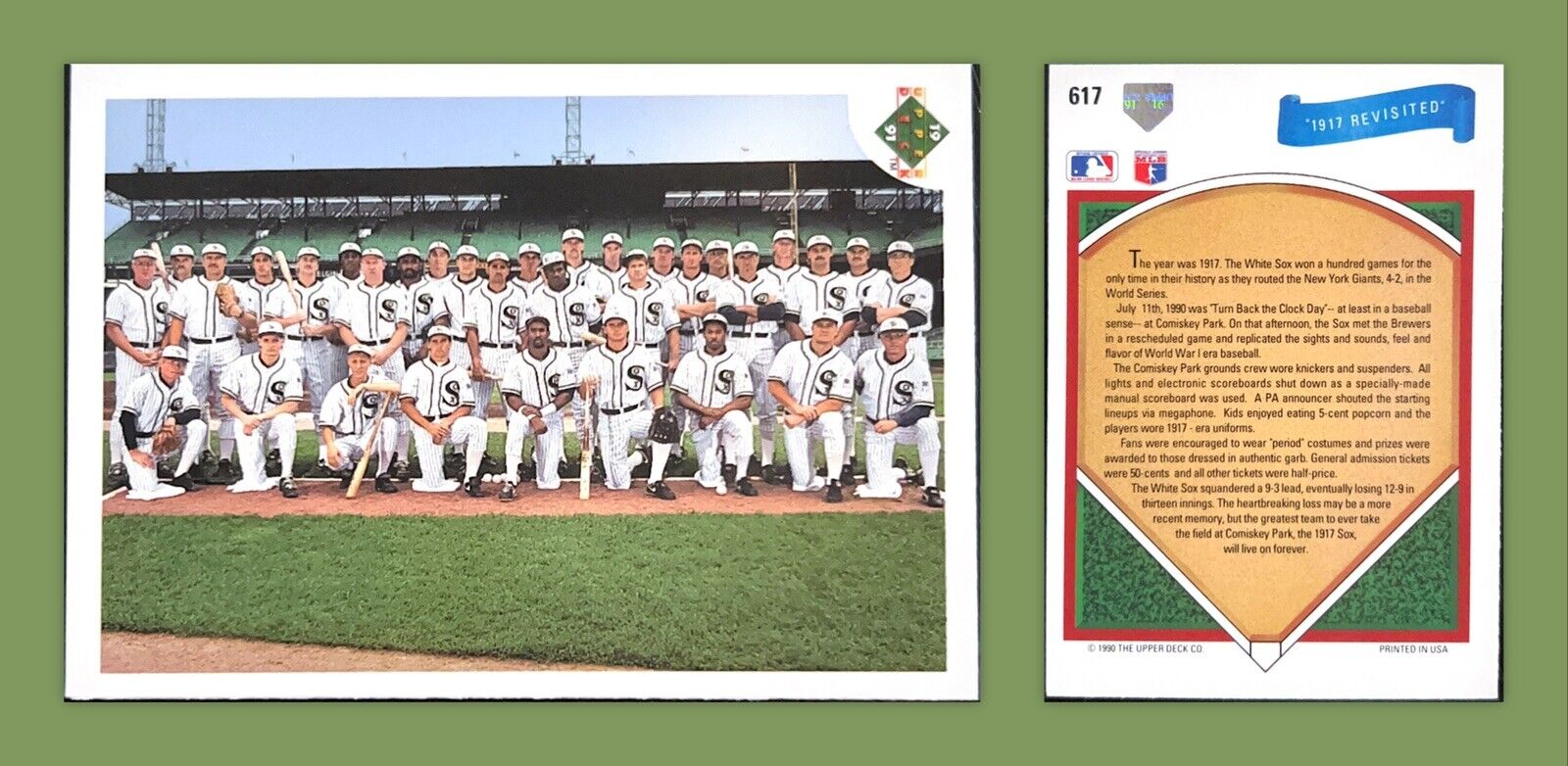The image features a horizontally rectangular composition against a sage green background, divided into two separate sections. On the left, the larger section showcases a white-bordered, full-color photograph of a 1917 Chicago White Sox baseball team. The players, dressed in white uniforms with a dark black "S" on the chest, are arranged in two rows: the front row kneeling on one knee and the back row standing. Some players hold baseball bats or gloves, while others have their hands folded over their chests. The background reveals the stadium's bleachers and light poles, extending skyward behind the team.

On the right side of the image is a vertically oriented baseball card. At the top left corner of the card, the number 617 is prominently displayed. Below this number is the National League Baseball logo. The card features a brown background designed to resemble a baseball diamond. A banner on the card reads "1917 Revisited," highlighting the historic significance of the year for the Chicago White Sox. Despite the presence of several lines of black text on the card, the font is too small to decipher. Overall, this composite presentation serves as a collector's display, combining a historic team photograph with a commemorative baseball card.